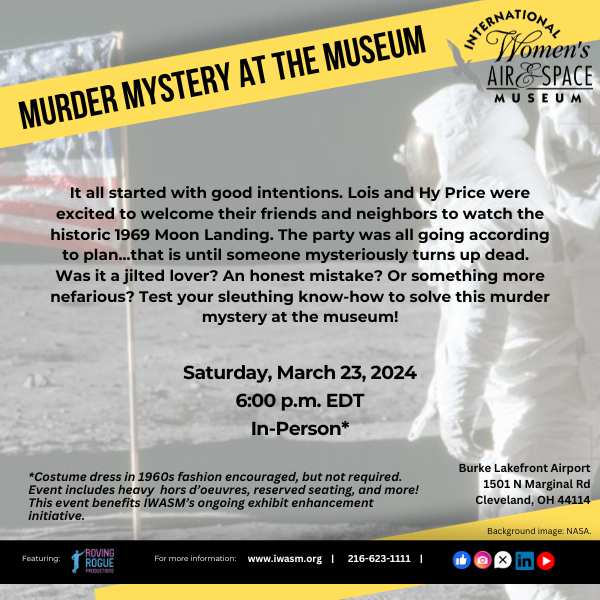This advertisement is for an event titled "Murder Mystery at the Museum," hosted by the International Women's Air and Space Museum. The poster merges color photography and graphic design, featuring a historic image of the 1969 moon landing. In the background, two astronauts in white spacesuits stand facing an American flag planted on the moon's surface. Across the top of the image, a yellow diagonal banner bears the event title in black text.

In the upper right corner, the museum's logo and name appear. Below, centered black text narrates the event's theme: "It all started with good intentions. Louis and High Price were excited to welcome their friends and neighbors to watch the historic 1969 moon landing. The party was all going according to plan. That is until someone mysteriously turns up dead. Was it a jilted lover, an honest mistake, or something more nefarious? Test your sleuthing know-how to solve this murder mystery at the museum." The event is scheduled for Saturday, March 23, 2024, at 6 p.m. EDT, to be held in person. 

Attendees are encouraged, but not required, to dress in 1960s fashion, with heavy hors d'oeuvres, reserved seating, and more included. This event supports the museum's ongoing exhibit enhancement initiative. Contact information includes the address Burke Lakefront Airport, 1501 N Marginal Road, Cleveland, OH 44114, and the website www.iwasm.org. Social media handles for Facebook, Instagram, Twitter, LinkedIn, and YouTube are also provided. Featuring Robin Rogue, the poster emphasizes that the background image is courtesy of NASA and highlights the supporting sponsors' logos in a black horizontal strip at the bottom.